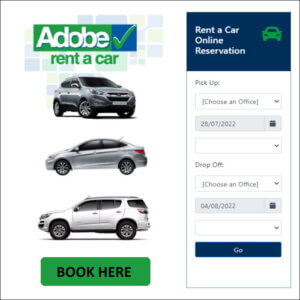The image displays a rental car website interface. At the top, there is a bar with options. Toward the right, the screen shows the Soitex logo along with the text "Rent a Car Online Reservation." 

Users can select "Pick Up" and "Drop Off" locations from a dropdown menu. The dropdowns display dates as "28/07/122" for pickup and "04/08/122" for drop off. 

To proceed, there is a prominent blue rectangle with the word "Go" on it. To the left, there is a section labeled "Adobe" with a green checkmark next to "Rent a Car." The background features a pattern of squares.

The interface also displays images of different cars available for rent. One is a grey car recognizable by its wheels, another is a silver car shown in profile, and there is also a large SUV. 

A green rectangle with black text that says "Book Here" is placed against a black-bordered section. The overall design is structured to guide users through the process of renting a car, with various elements emphasizing its functionality and user-friendliness.